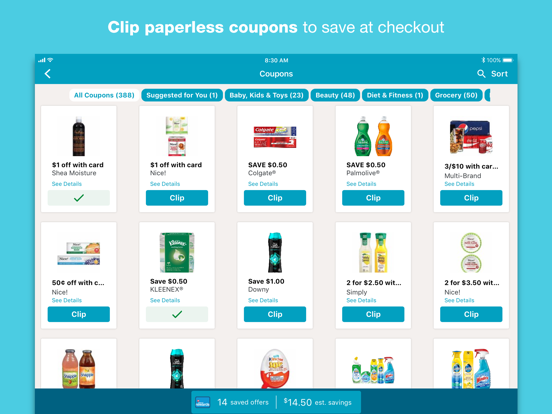**Image Caption:**

At the top of the image, a message in white text reads, "Clip paperless coupons to save at checkout." The time is displayed as 8:30 a.m., followed by the word "Coupons." The categories under "All Coupons" include suggested sections for "You," "Baby," "Kids and Toys" (23 offers), "Beauty" (48 offers), "Diet and Fitness" (1 offer), and "Groceries" (50 offers).

The image prominently features several coupon deals, including:
- $1 off with card for Shea Moisture shampoo, which is visually represented by a bottle of shampoo.
- $1 off with card for Nice products.
- Save 50 cents on Colgate products.

Customers have the option to "Clip" these coupons by clicking the word "Clip" next to each deal. Additional deals include:
- 50 cents off two bottles of Palmolive dish detergent.
- Three sodas for $10 with card.
- 50 cents off Nice products.
- Save $1 on Downy.
- Two Simply Orange juices for $2.50.

The bottom row of the image showcases further offers, including Snapple drinks, another container of Downy Unstoppables, Kinder Joy, and various house cleaning products. The accumulated savings from clipping these offers totals 14 saved offers and an estimated savings of $14.50.